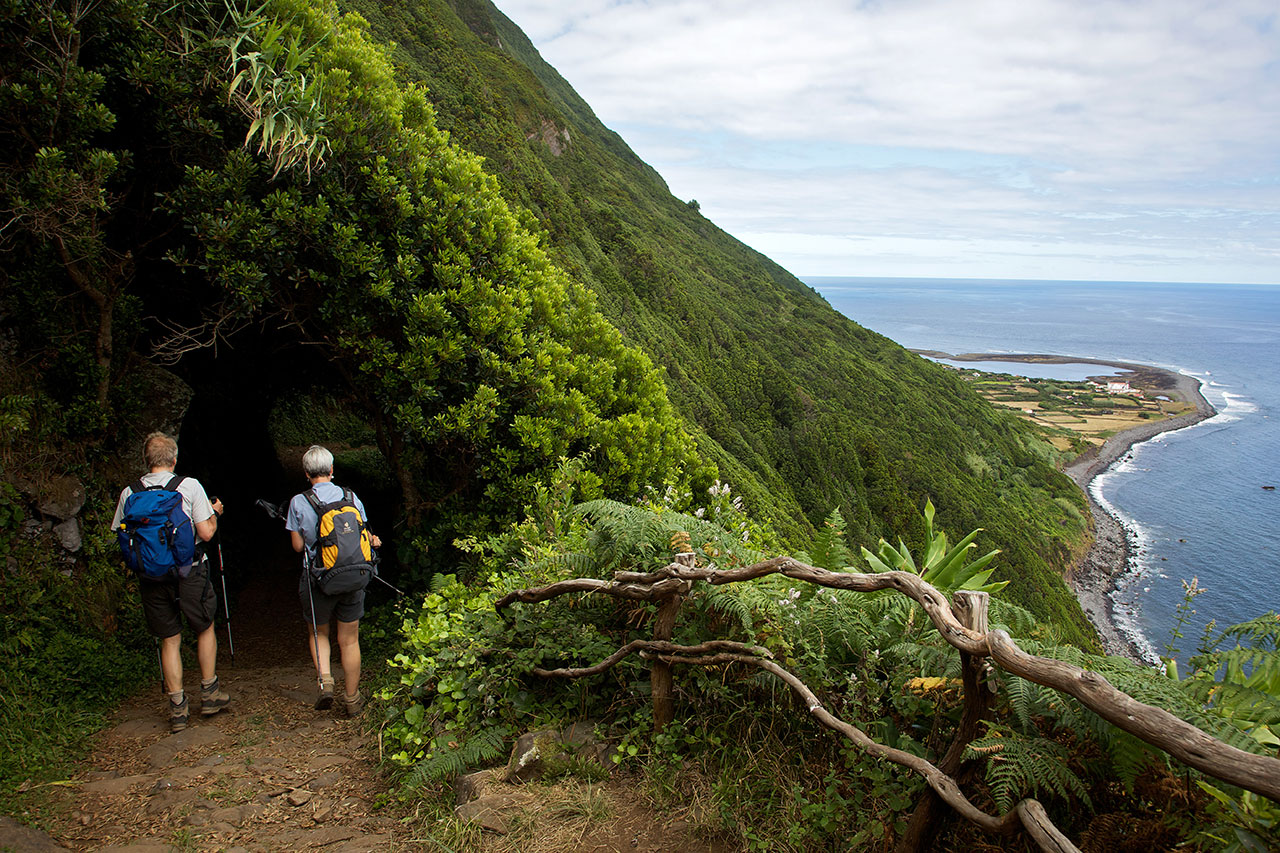The photograph captures an outdoor scene of a couple, likely in their late 50s or early 60s, embarking on a hiking adventure. They have their backs turned to the camera and are equipped with hiking sticks, backpacks, and are dressed in T-shirts, black shorts, and hiking boots. The couple is positioned at the bottom left corner of the image, heading towards a dense, cave-like forested area where the trees form a dark, tunnel-like canopy.

The setting is a lush, green, mountainous terrain that slopes down towards a coastline. To the right of the frame, the ocean is visible, with a long beach and possibly some farmland or houses in the distant background. The area appears to be an island, surrounded by water. A natural fence made of twisted, gnarly tree branches runs parallel to the path, possibly to prevent hikers from falling due to the significant elevation. The scene is bright and sunny, highlighting the vibrant green foliage that envelops the trail.